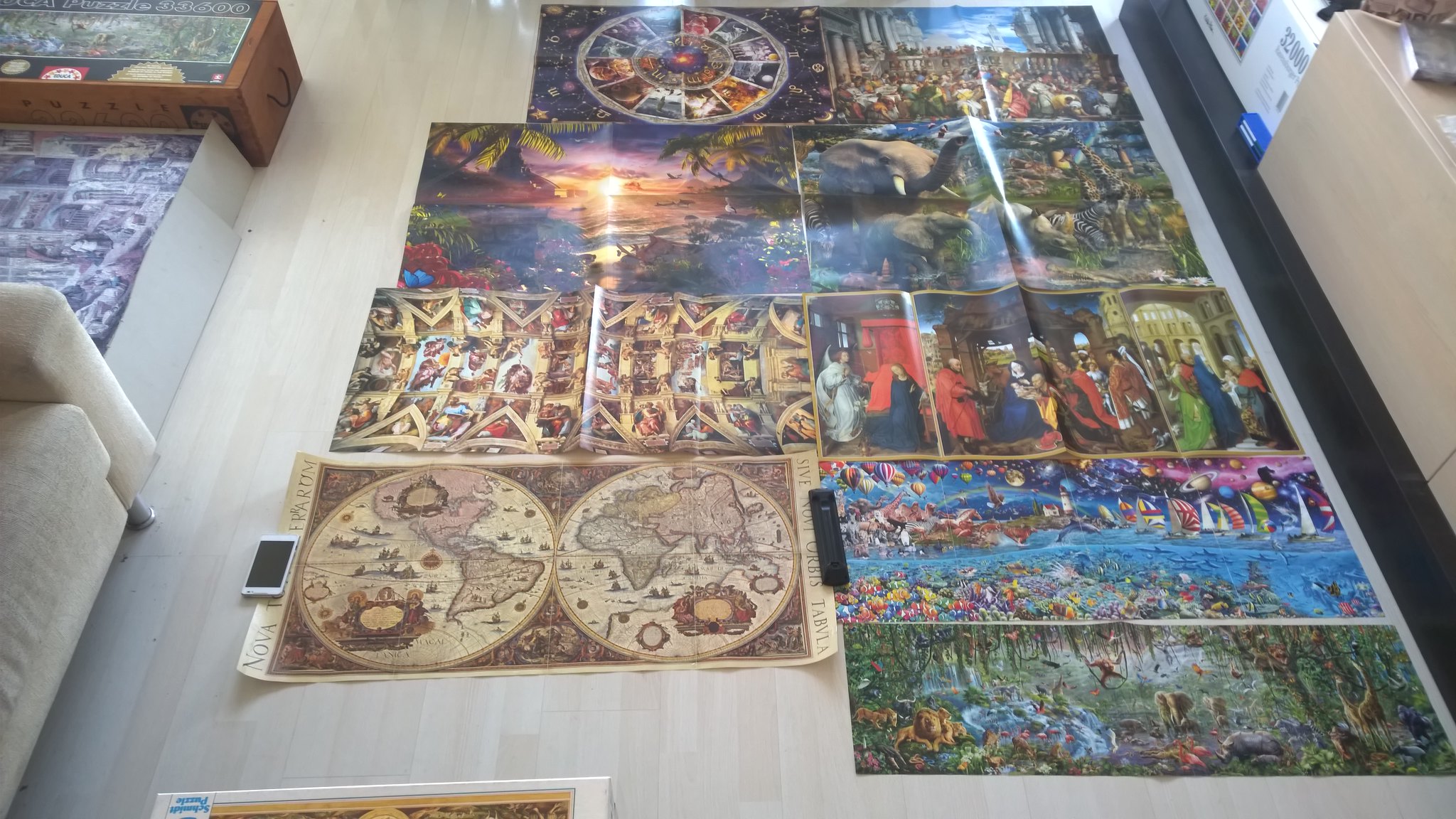The color photograph, taken from above, showcases a collection of vividly colored artistic prints and posters arranged flat on what appears to be a brand new, light-colored wooden floor. In the left-hand portion of the image, a beige couch and a table intrude slightly, while on the right, a cardboard box filled with items can be seen alongside a piece of furniture with a black border. Among the prints, a map lies prominently in the bottom left-hand corner. The other eight prints, exhibiting slight creases, resemble professionally created Renaissance and fantasy paintings, embodying various themes from a tropical sunset with palm trees and a glaring sun, to African wildlife scenes featuring elephants and zebras, and even an array of planets in a celestial setting. Intriguingly, one poster near the edge of the couch has a phone resting on it, while a remote control sits centrally atop another. The scene reflects a blend of meticulous artistic detail and casual domestic arrangement.